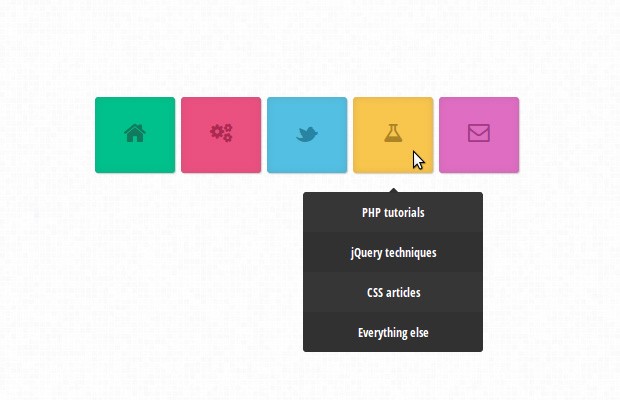The image features a section of a webpage displaying a horizontal row of five square icons with rounded corners, each uniquely colored and corresponding to different menus. The sequence from left to right includes a green square representing the home menu, a magenta (or red) square with gears indicating the settings menu, a light blue square reminiscent of the Twitter logo, a golden-yellow square depicting a science beaker with a drop-down menu, and a purple square with an envelope icon for email. The drop-down menu under the golden-yellow beaker icon contains options for PHP tutorials, jQuery techniques, CSS articles, and additional resources. The entire user interface is set against an off-white backdrop, and a white mouse cursor is shown hovering over the golden-yellow icon, revealing the drop-down menu.